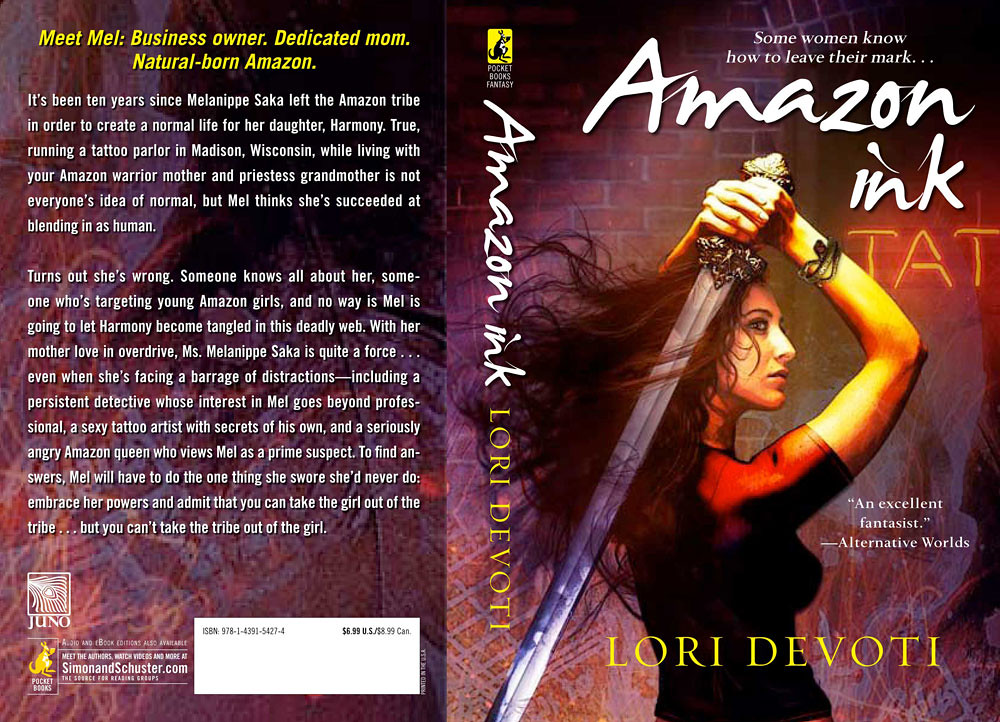This is an image of an unfolded book cover for "Amazon Inc." by Lori Devoree. The front cover, on the right side, features a dramatic profile of a woman with long, dark hair flowing around her as she stands in front of a brick wall. She holds a jewel-encrusted sword behind her head with both hands. The top of the cover reads, "Some women know how to leave their mark," while the author’s name, Lori Devoree, is prominently displayed below. There's an endorsement stating, "An excellent fantasist," by Alternative Worlds. The back cover introduces the protagonist with the text, "Meet Mel: business owner, dedicated mom, natural born Amazon," followed by more details about the character, Melanippe. The book is priced at $6.99 in the US and $8.99 in Canada and is published by Simon and Schuster. The ISBN number is also visible on the back cover.